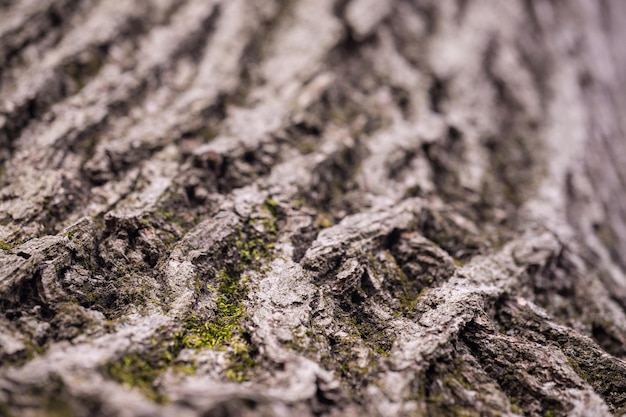This is a highly detailed, close-up image of a tree trunk, showcasing its textured bark with intricate grooves about an inch deep. The bark exhibits a range of earthy tones, including shades of brown, gray, and off-white, with patches of weathered, eroded bark fibers. A horizontal line, possibly a rope or a natural feature of the bark, runs across the image. A vibrant lime-green moss grows vertically within the grooves and cracks of the bark, particularly prominent in the middle and toward the bottom left side. This natural mesh-like pattern is further accentuated by faint hints of green throughout the bark, suggesting the presence of additional lichen or moss. The image has a somewhat blurred top right corner, indicating depth and focusing on the clarity of the bottom half. The setting is clearly outdoors, likely photographed during the daytime, capturing the dynamic textures and colors of the tree trunk.